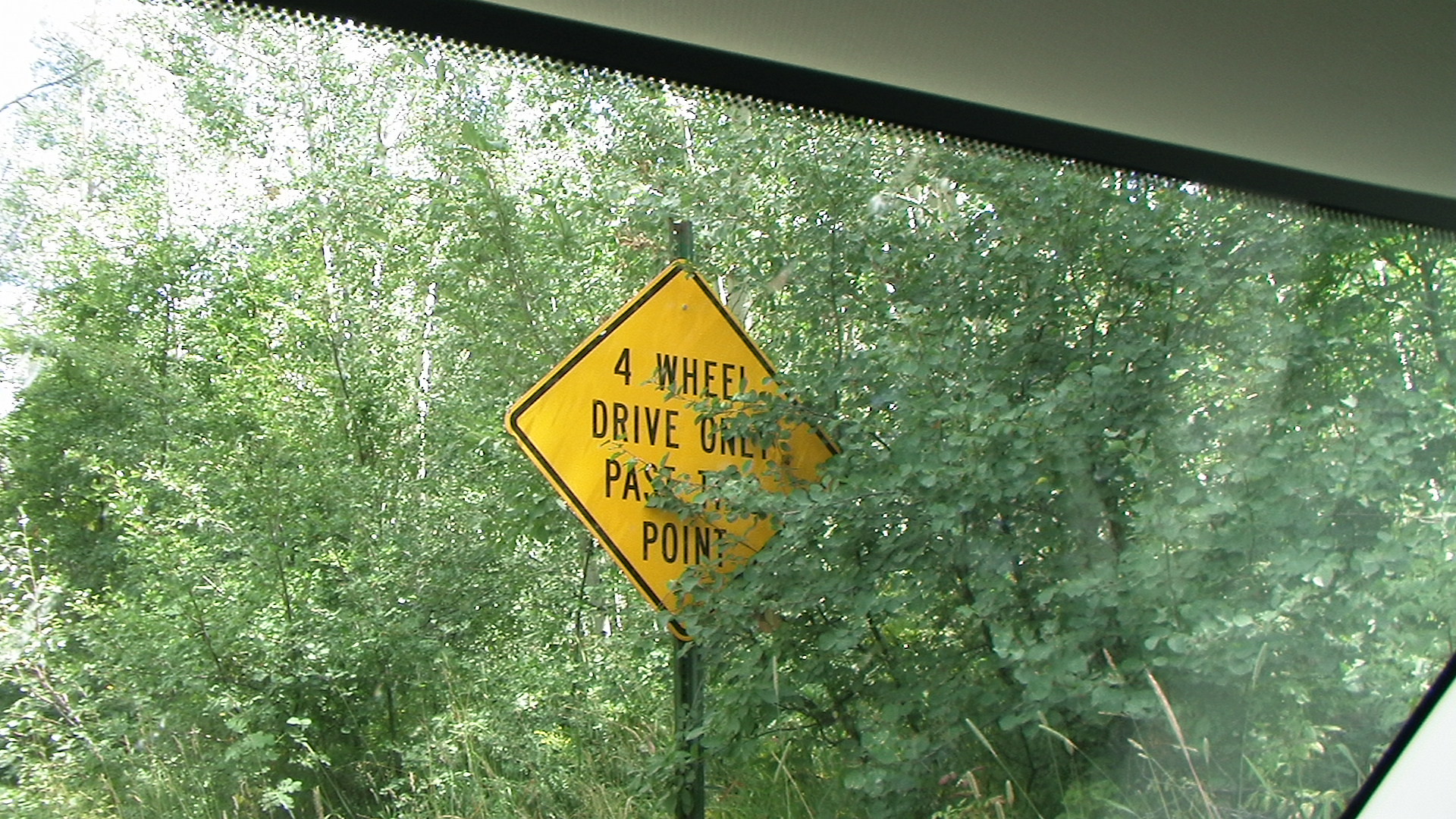The image captures a view through the windshield of a large car. The scenery visible through the windshield predominantly features a dense, tree-filled forest with abundant greenery. In the midst of the verdant landscape, a sign is visible, which reads "Four Wheel Drive Only." However, the sign is partially obstructed by a branch, particularly obscuring parts of the text around the word "Only." The windshield of the car has a tinted white gradient at the top and is edged with a black trim, adding defined borders to the view.